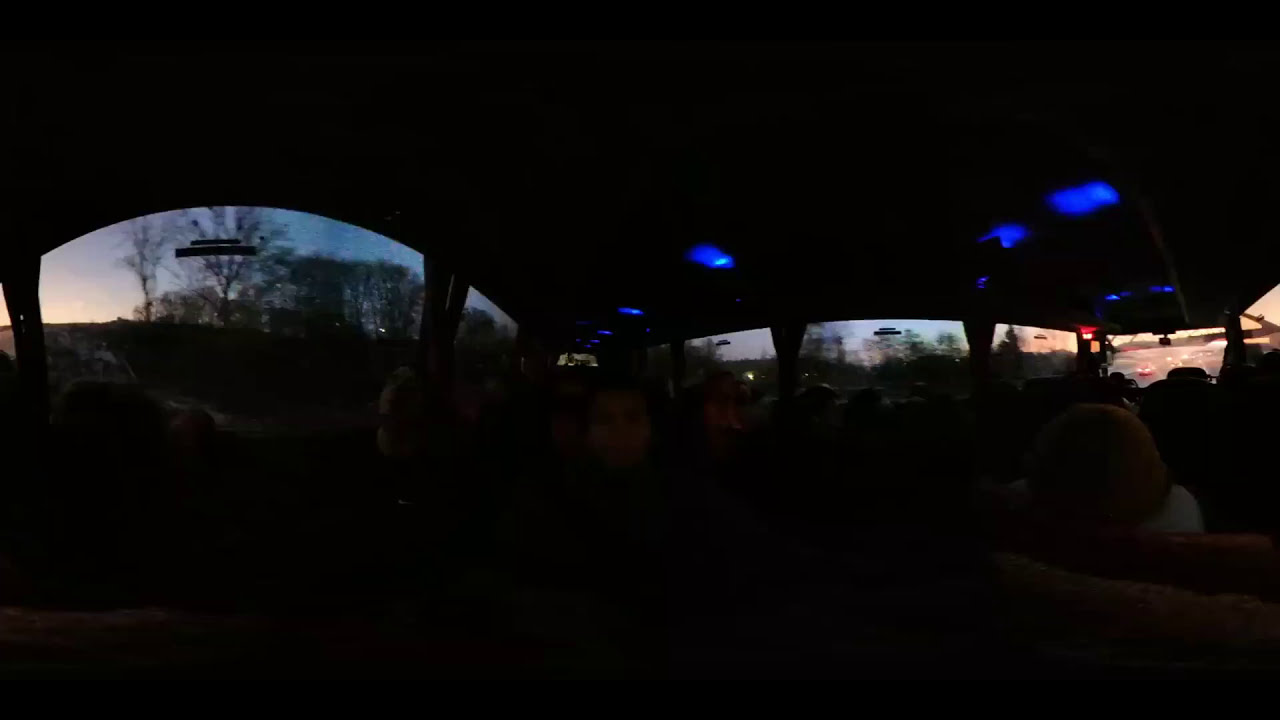In this dark, panoramic image, we see the interior of a bus filled with seated passengers, their features obscured by the lack of light. The focal point is a woman at the center, with people sitting on either side, many looking into the camera. The bus is semi-lit by dim blue lights embedded in the roof, contributing to the overall low visibility. The windows along the sides offer glimpses of the outside, where it's late in the evening, evidenced by the dusky sky and the setting sun. Through the left windows, leafless trees can be seen, while the right side reveals a parking lot or road with some cars visible. There are no visible text elements in the image. The color palette includes shades of black, gray, tan, red, white, blue, and orange, with the scene cast in deep shadow, enhancing the mysterious atmosphere.